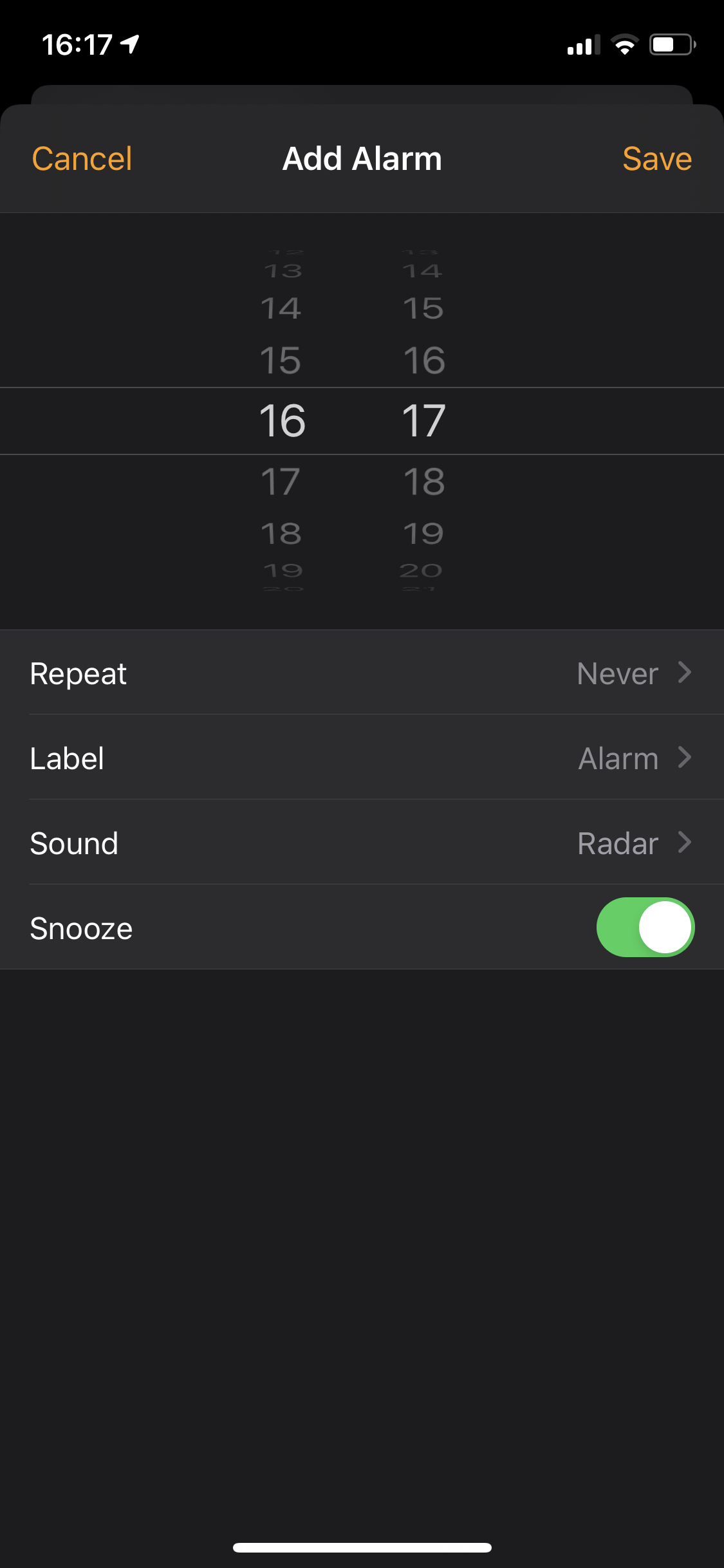Screenshot of the "Add Alarm" Setting on a Smartphone

The image features a screenshot showcasing the "Add Alarm" setting interface on a smartphone with a black background. The top section of the screen includes a lighter gray banner. On the left side in orange text is the option to "Cancel," and on the right side in the same orange text is the option to "Save." Centrally located between these options is the "Add Alarm" title in white text.

Beneath this banner, there is a time selection section displayed in the form of rotating wheels. The currently selected time is shown as 16:17, with the numbers 16 and 17 prominently displayed in the middle row. Above these numbers are smaller increments: 13, 14, 15 to the left and 14, 15, 16 to the right. Below the selected time, the increments continue with 17, 18, 19 to the left and 18, 19, 20 to the right.

Further down, there is a list of additional alarm settings including:
- "Repeat" set to "Never"
- "Label" set to "Alarm"
- "Sound" set to "Radar"
- "Snooze" feature, which is turned on.

To the right of the "Snooze" option is a green and white toggle switch indicating that snooze is enabled.

Additionally, the status bar at the top of the phone screen shows the device has three out of four bars of cellular signal, two bars on the Wi-Fi signal, and approximately 55-60% battery charge.